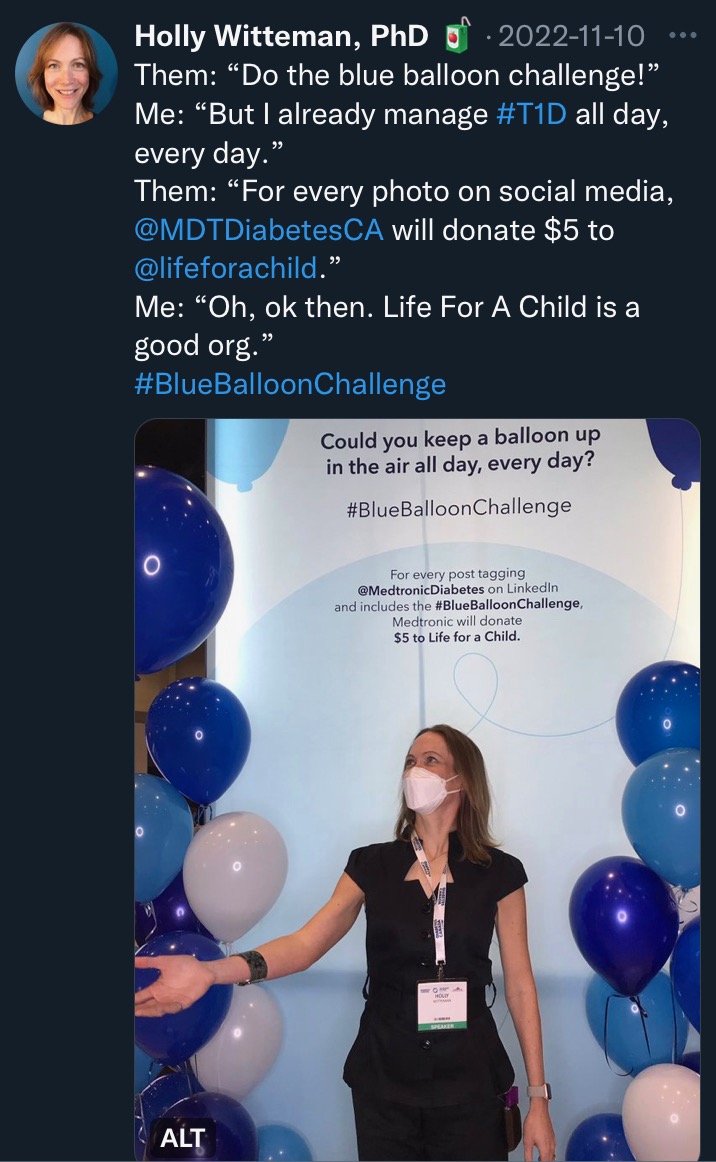The image features a social media post by Holly Whitman, Ph.D., dated November 10, 2022. The text at the top introduces the "Blue Balloon Challenge," encouraging participation to support Diabetes awareness. It mentions that for every social media post featuring a blue balloon and tagging @mdtdiabetes.ca, the company will donate $5 to Life for a Child, a charitable organization. Below the text, a photo captures Holly Whitman, wearing a mask, surrounded by a mix of blue and white balloons. The overlay on the photo challenges viewers with the question, "Could you keep a balloon up in the air all day, every day?" accompanied by the hashtag #BlueBalloonChallenge.